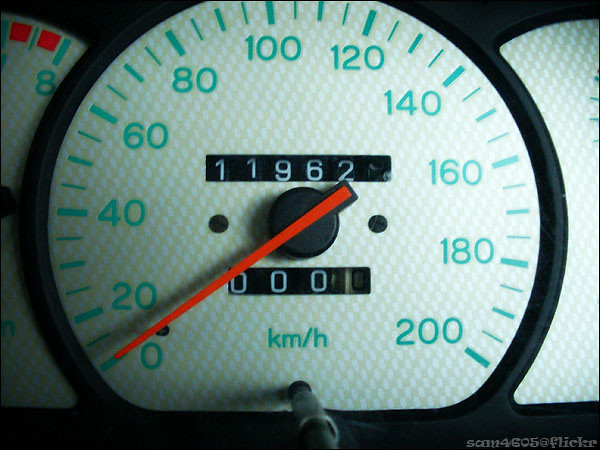This photograph captures the intricate details of a car's dashboard, featuring a cluster of various gauges and indicators. The centerpiece is an odometer calibrated in kilometers, ranging from 0 to 200. The odometer specifically highlights a total mileage of 119,620 kilometers, while the trip meter is reset to zero. The dashboard's background has a linen-like texture, accented with fluorescent green numerals and markings. Two screws are visible, securing the gauge panel. A prominent red needle indicates the current speed.

Flanking the central speedometer are two additional gauges. The right gauge is partially visible, showing only a few green lines—possibly indicating the fuel level. The left gauge displays an '8', alongside a series of green lines and red boxes, and also contains a visible screw on the side. The overall framing and outlines of the dashboard are in black, complementing the intricate design elements. A small black button is seen on the front, used to reset the trip meter, adding a functional touch to this well-used yet meticulously maintained control panel.